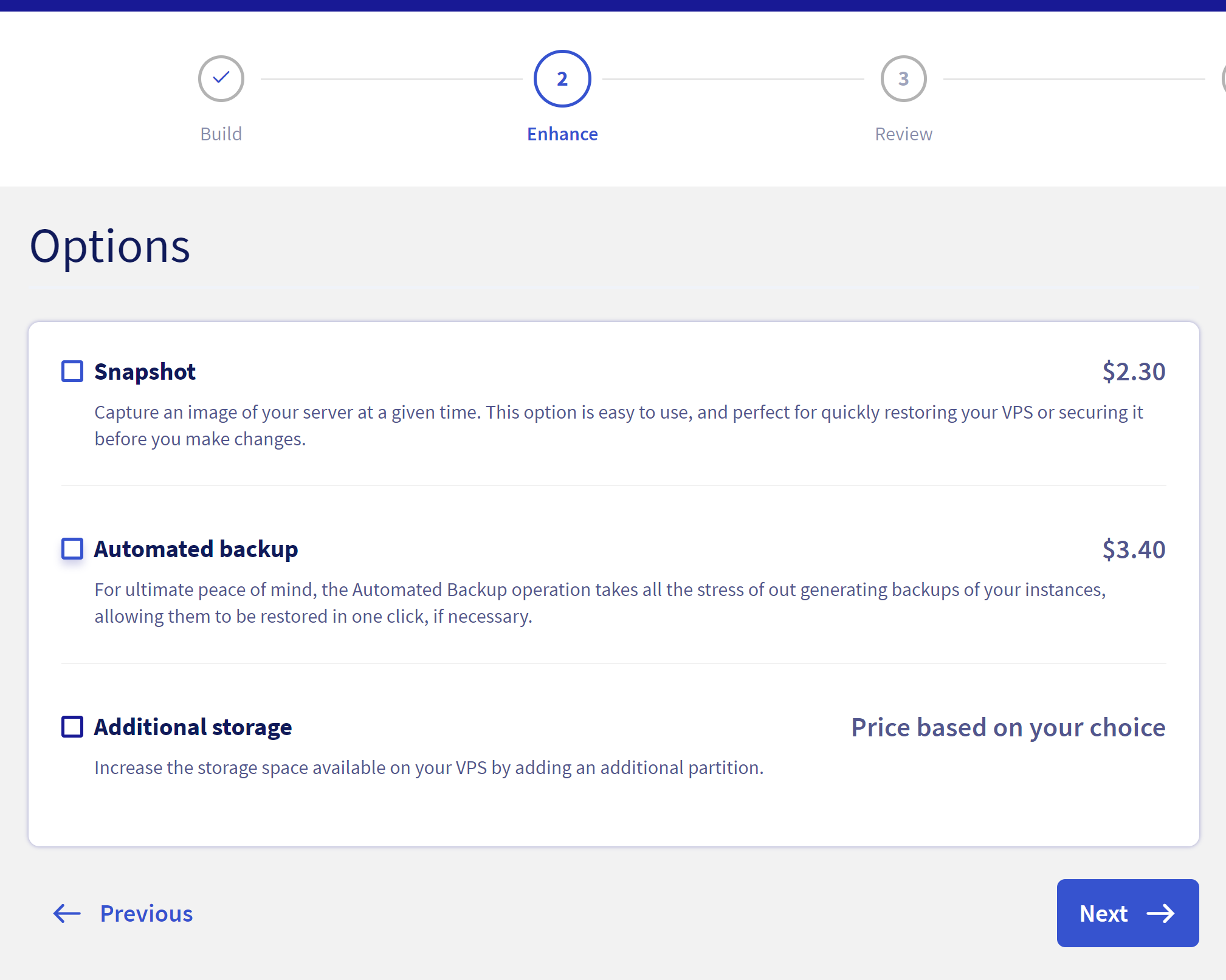In the top right corner, there is a blue horizontal bar with a grey circle inside it labeled "Checkpoints and Bill." Within this circle is the number "2" in blue. Below, the blue bar contains several elements: "Enhanced," "Review," and a series of lines. There is a bold blue text label that says "Options."

Beneath "Options," there is a box labeled "Not Tracked" with two sections inside it. The first section is labeled "Snapshot" and displays a price of "$2.30." This option is described as capturing images at a given time, making it easy to quickly restore your VPS or secure relevant changes.

The second section, also labeled "Not Tracked," states "Automated Backup" and echoes the price of "$2.30." This option offers an automated backup feature, which simplifies the generation of records for your instances, allowing them to be restored in one click to a state of 340.

Additionally, there's an option to increase the storage space available on your VPS by adding any additional partition of your choice. 

Towards the bottom, a left-pointing arrow labeled "Previous" and a blue checkmark are visible. 

This collection of options and information is presented within a website interface designed with various text types and displayed in squares with rounded edges.